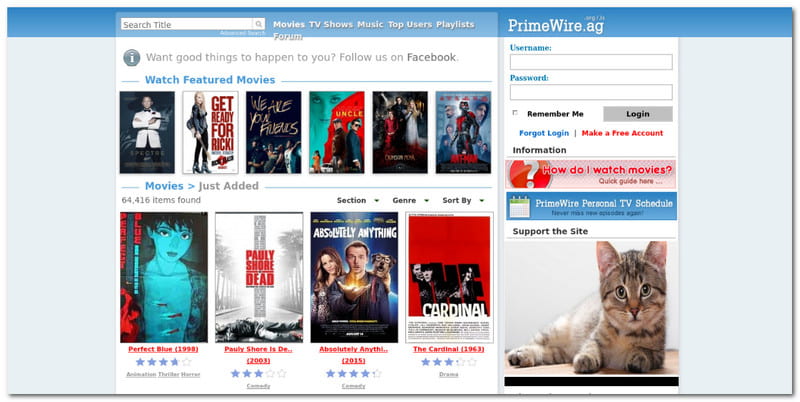The screenshot showcases the homepage of the Primewire.ag website, a platform dedicated to streaming movies, TV shows, and music. The top section features a light blue navigation bar with the Primewire.ag logo on the left and a login section on the right, prompting users to enter their username and password to access their accounts. Adjacent to the logo, a search bar invites users to "search titles," and next to it are categories listed in white font: Movies, TV Shows, Music, Top Users, and Playlists.

Beneath the navigation bar, there's an advertisement encouraging users to join PrimeWire through Facebook. Below the ad, the page displays a series of clickable thumbnails, each representing different movies available for streaming. Towards the bottom right corner of the page, a small image of a cat is captioned "Support the site," indicating a request for donations, suggesting that the website operates on a low budget.